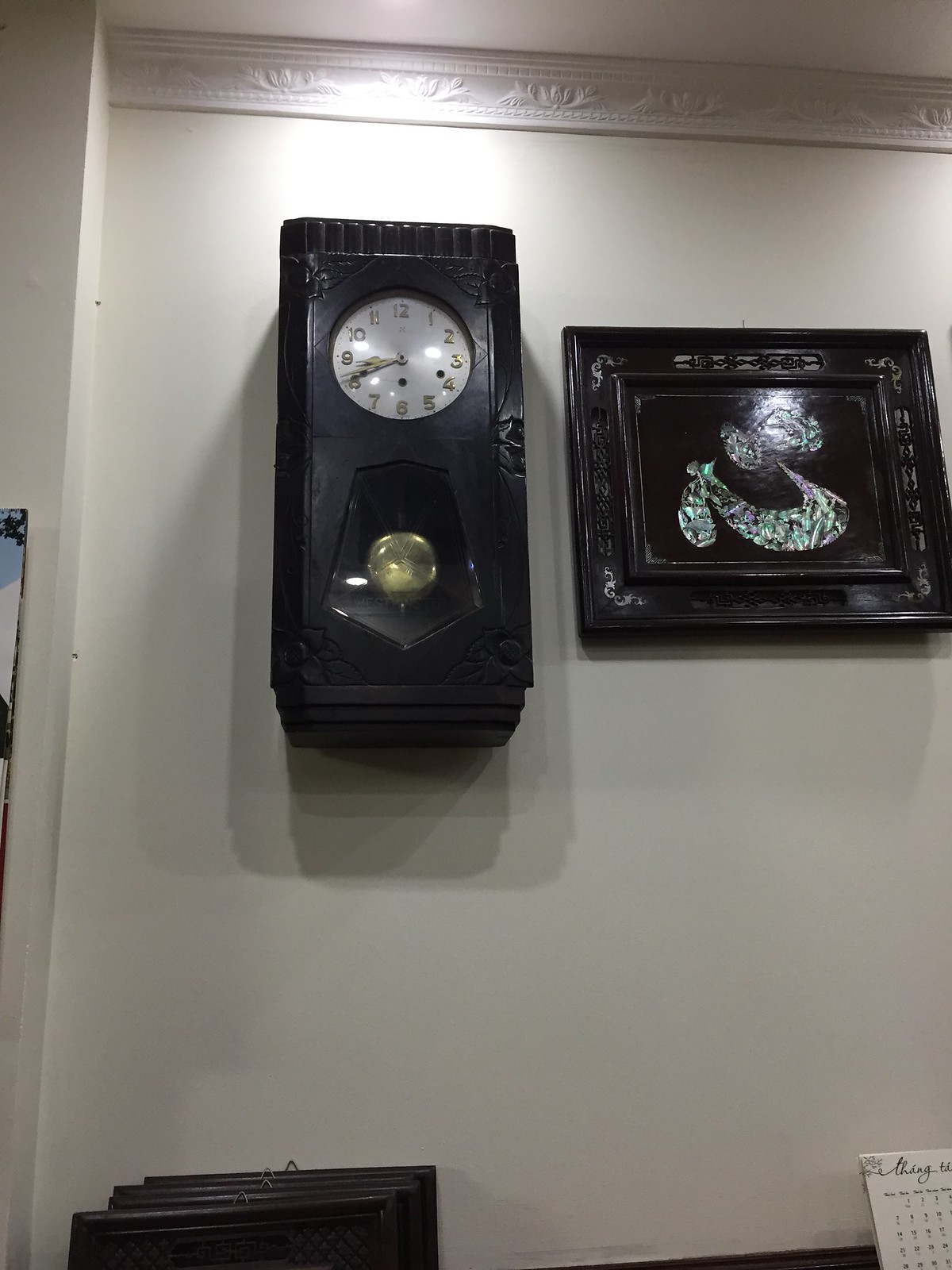This color photograph features a plain white wall adorned by two distinct items: a clock and an artwork. The clock, prominently displayed, has a dark wood casing that contrasts with its white dial. Gold numerals and hands add an elegant touch to the clock, which shows the time at approximately 8:40. The clock face is protected by a glass covering, evident from the reflections visible on its surface. Adding to its ornamental design, the clock showcases a large, round gold pendulum encased in glass at its bottom.

To the right of the clock hangs a piece of artwork framed in a black, intricately carved frame. The art itself is somewhat ambiguous but appears to be a mosaic created from pieces of mother-of-pearl, adding a touch of iridescence and complexity to the composition. Together, these elements create a refined and intriguing wall display.